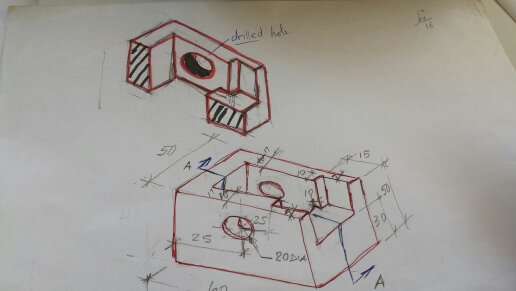The image features a photograph of a technical design sketched on a large white sheet of paper, possibly printer paper, which appears to be laid out on a drafting table or perhaps hung on a wall. Prominently, there is an L-shaped or half-rectangle figure near the top of the page with a labeled "drilled hole," annotated in blue pen or marker with a line pointing to it. This figure is intricately drawn in dark blue or black marker, along with some red detailing. Below this, a more complex, three-dimensional structure composed of interconnected rectangles can be seen. This structure, also unlabeled but surrounded by numerous measurements and annotations, hints at real-world construction dimensions. The back side of this figure is marked with an "A", further detailing the design's assembly or orientation. The presence of various numbers and measurements suggests this could be an architectural or engineering schematic intended for building an object, potentially made of wood.